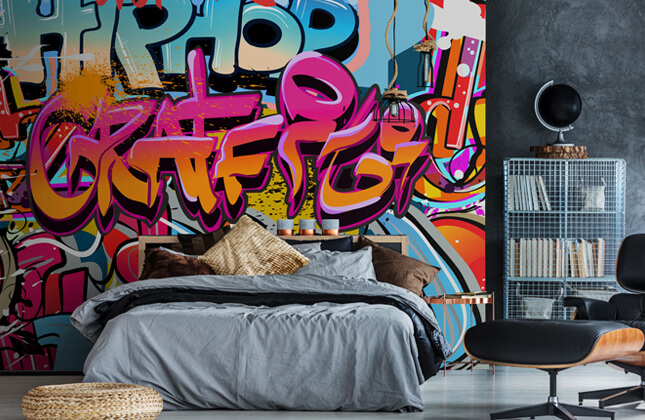The image portrays a bohemian studio bedroom, dominated by an expansive graffiti mural that covers much of the back wall. The dynamic artwork, bursting with vibrant colors like pink, blue, and orange, features bold lettering that reads "Hip Hop Graffiti" in a comic-style print. The text is vividly outlined in black and accentuated with a pink-to-orange gradient over an array of colorful shapes. Below this eye-catching mural sits a double bed adorned with light gray covers, a dark blanket, and an assortment of pillows in various shades of brown. To the right of the bed, a modern black lounging chair is accompanied by a matching leather footstool. A wire-metal bookshelf adorned with books stands nearby, crowned with a black globe. The room’s eclectic and artistic design is further enhanced by a light brown wicker basket positioned at the foot of the bed, adding a touch of rustic charm to the otherwise contemporary space.